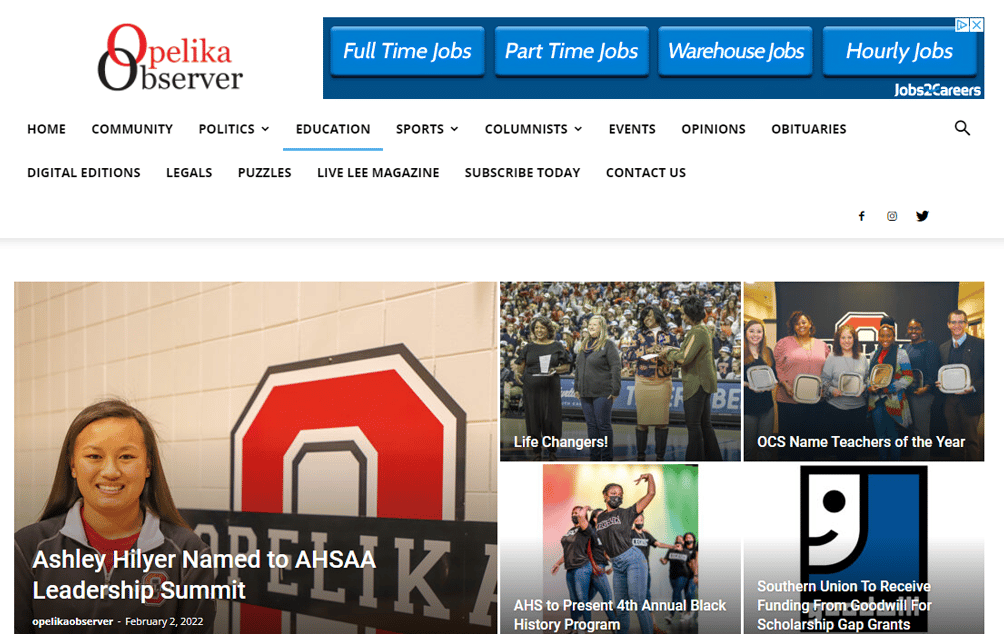The screenshot displays a section of a website with a predominantly white background. Positioned in the upper left corner, "Opelika" is written in red text, and "Observer" is in a darker color, likely black or blue, with the two O's from each word intertwined like rings. To the right are four action buttons labeled "Full-Time Jobs," "Part-Time Jobs," "Warehouse Jobs," and "Hourly Jobs." These buttons are set against a blue backdrop, under which it reads "Jobs to Careers" in white text.

Below the action buttons is a navigation bar with menu items listed from left to right: "Home," "Community," "Politics" (with a pull-down arrow), "Education" (highlighted with a blue line link), "Sports" (with a pull-down arrow), "Calmness" (possibly a typo for "Columns," also with a pull-down arrow), "Events," "Opinions," and "Obituaries."

Further down, there is another navigation line featuring links to "Digital Editions," "Legals," "Puzzles," "Live.ly Magazine," "Subscribe Today," and "Contact Us." On the far right side of this line, icons for Facebook and Twitter are displayed.